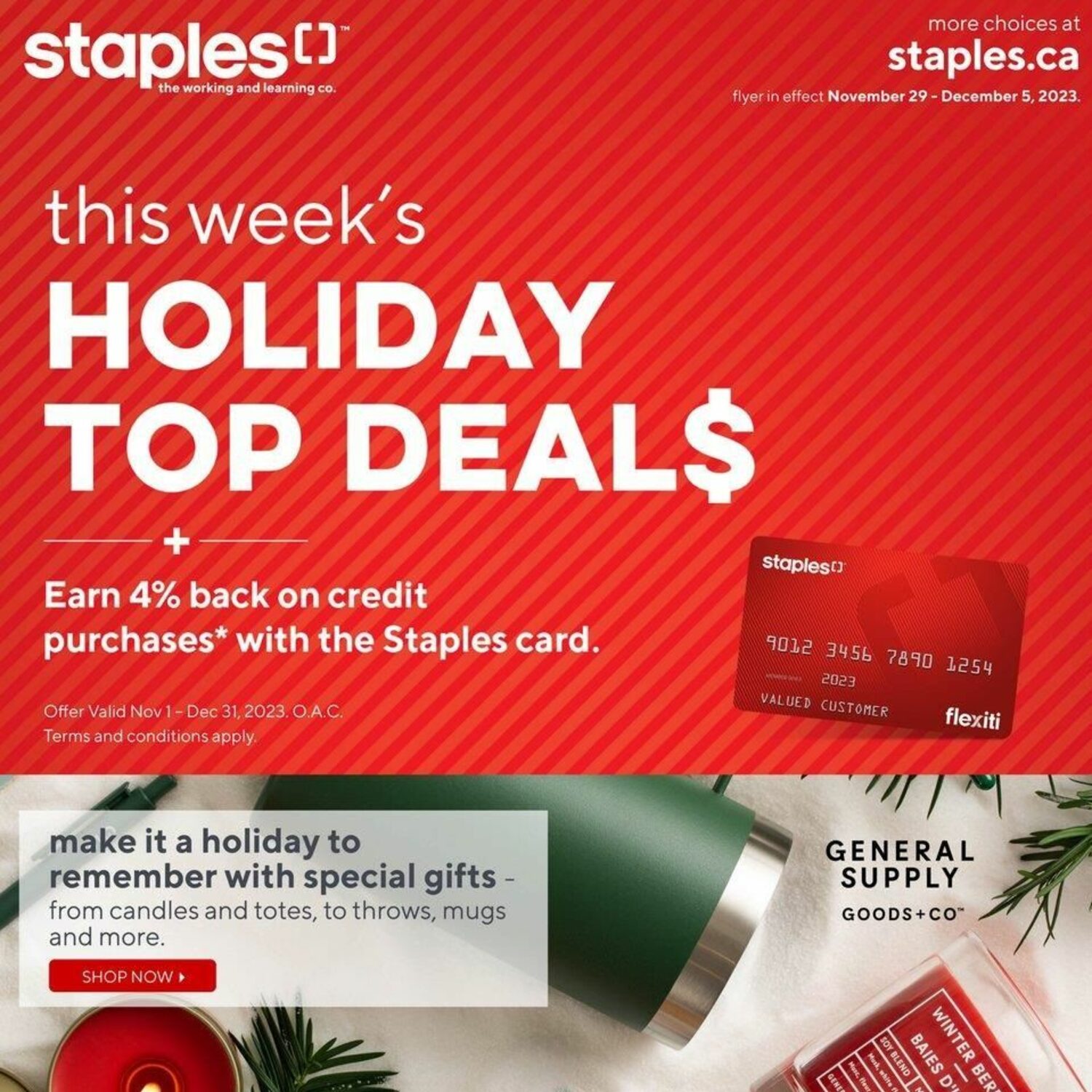The image in question is a promotional flyer for Staples, prominently featuring the company logo in the top left corner, accompanied by the tagline "The Working and Learning Company." To the right, the tagline highlights "more choices at staples.ca," indicating the Canadian branch of the retailer. The flyer, valid from November 29th to December 5th, 2023, has a bold design with the top 75% dominated by a red background with diagonally descending stripes in alternating shades of red.

Centered in this red section, the promotional text reads "this week's" in non-bolded, lowercase font. Beneath it, "HOLIDAY TOP DEALS" is featured in bold, all caps, white text, where the 'S' in 'DEALS' is represented by a dollar sign ($). The headline is complemented by a plus symbol (+) and the text "Earn 4% back on credit purchases," followed by an asterisk indicating the need for a Staples card. Further explanation provided by the asterisk notes, "Offer valid November 1st through December 31st 2023. OAC terms and conditions apply."

The flyer conveys that Staples offers more than just office supplies, including special holiday gifts ranging from candles and totes to throws, mugs, and more. A selection of these gift items is visually showcased near the bottom of the flyer, featuring a festive mug and a candle, suggesting thoughtful gift options for the holiday season.